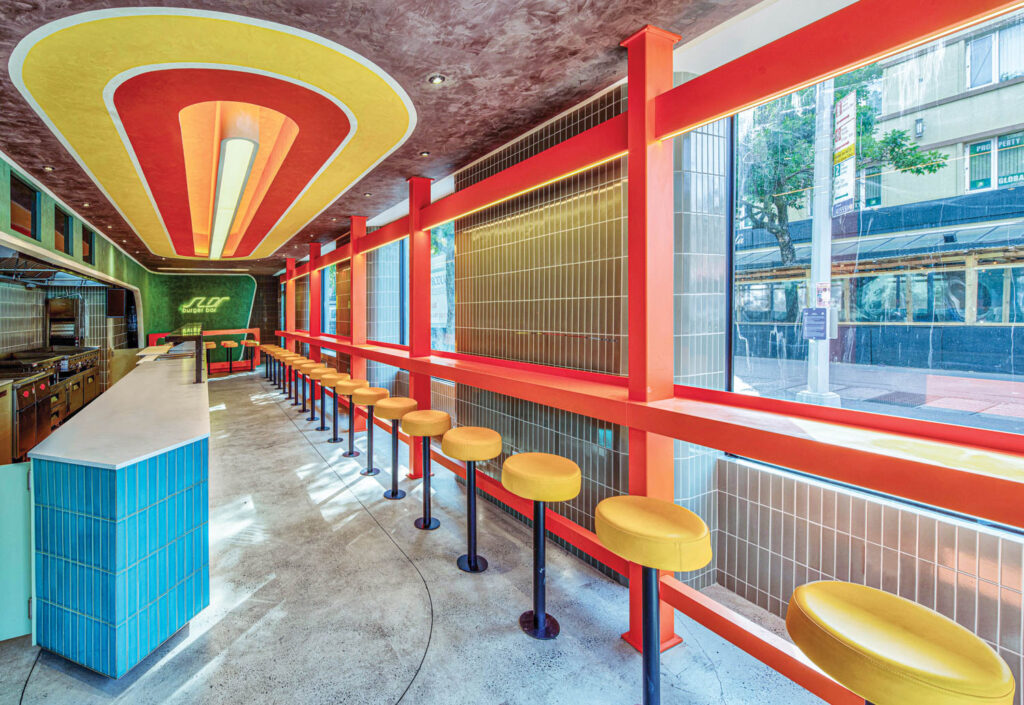This vibrant color photograph captures the bustling interior of a diner located on a busy main street, flooded with natural light through large windows. The diner combines modern and vintage elements in its decor, predominantly featuring a palette of red, orange, and yellow. Along the length of the large rectangular space, there are backless barstools with orange-yellow tops and black bases, lined up against a lengthy countertop facing the windows, offering a view of the lively street outside. The window sills and the ceiling exhibit a striking red hue, adding to the colorful ambiance. The ordering counter is distinguished by a white countertop with a blue base, contrasting with the green backdrop wall behind it. The ceiling, adorned with space-themed graphics, enhances the unique atmosphere of this city diner, which exudes a nostalgic yet modern charm.